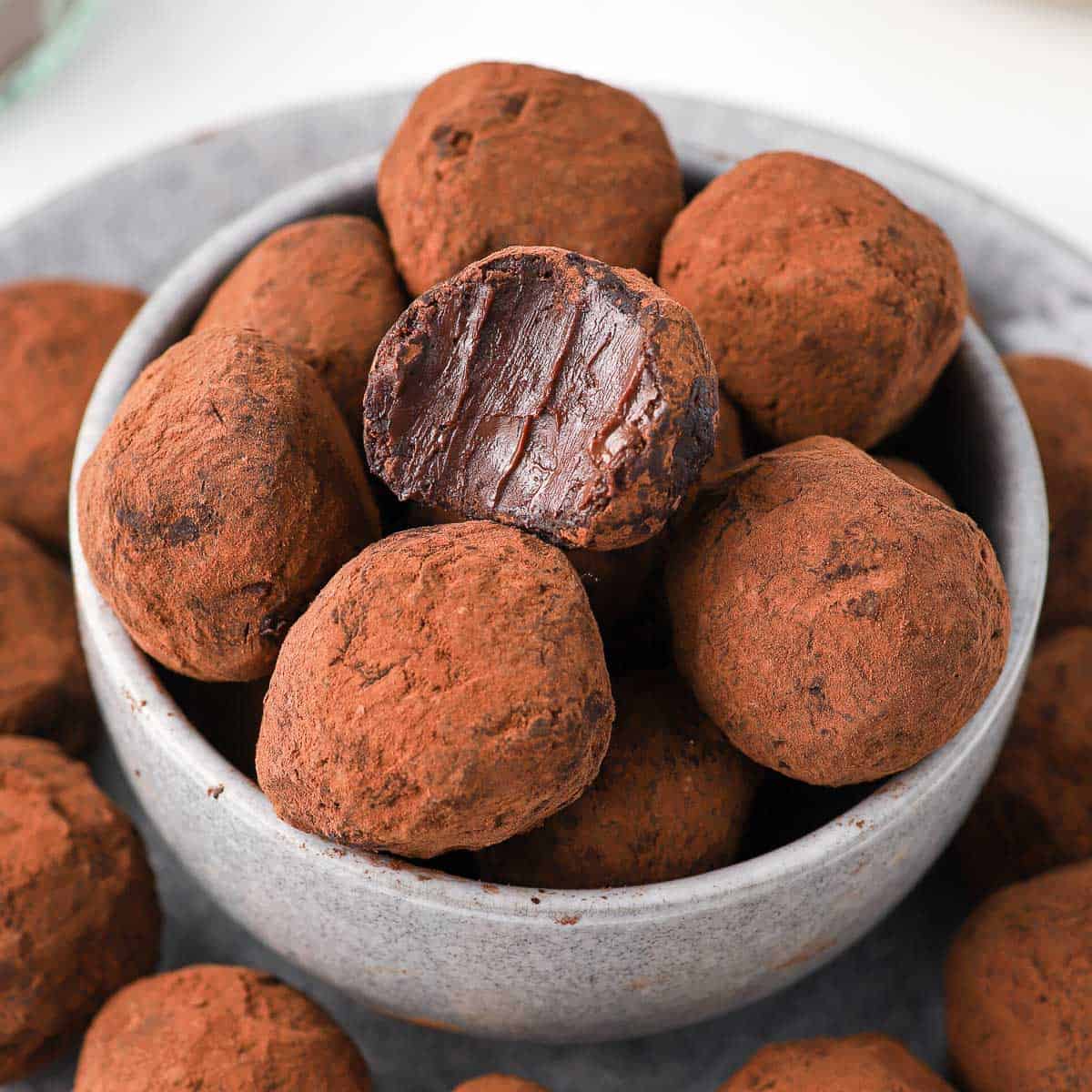This is a professional square-format color photograph, likely taken indoors, featuring an aesthetically arranged gourmet chocolate truffle display. At the center of the image, a light gray, speckled stone bowl is filled with round, hand-rolled chocolate truffles dusted in a brick-red cocoa powder. Prominently, one truffle in the bowl has a bite taken out, revealing a rich, dark brown chocolate fudge interior. The bowl rests on a matching light gray speckled stone plate, with additional truffles encircling it on the plate's surface. This carefully composed and high-quality food photography piece emphasizes the luxurious, artisanal nature of the chocolates and the elegant, likely expensive, ceramic serving ware.